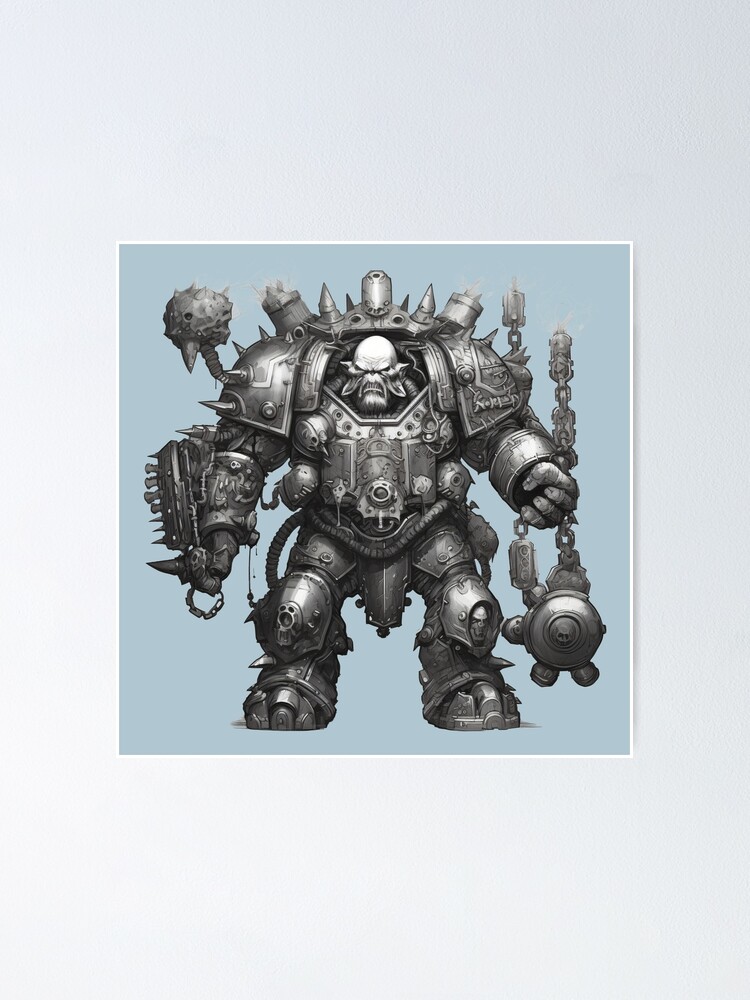The image depicts a computer-generated, battle-ready goblin man clad in full heavy, spiked armor, emphasizing his large, bald head with a pronounced forehead, giving him an alien-like appearance. He stands menacingly with a mace in his left hand and a loop-shaped chain in his right. His armor, a dark gray with black accents, covers him from head to toe, featuring various spikes and intricate armory, exuding a medieval and monstrous vibe suggestive of a video game character. The background is a solid light grayish-blue, spotlighting his imposing, otherworldly presence.